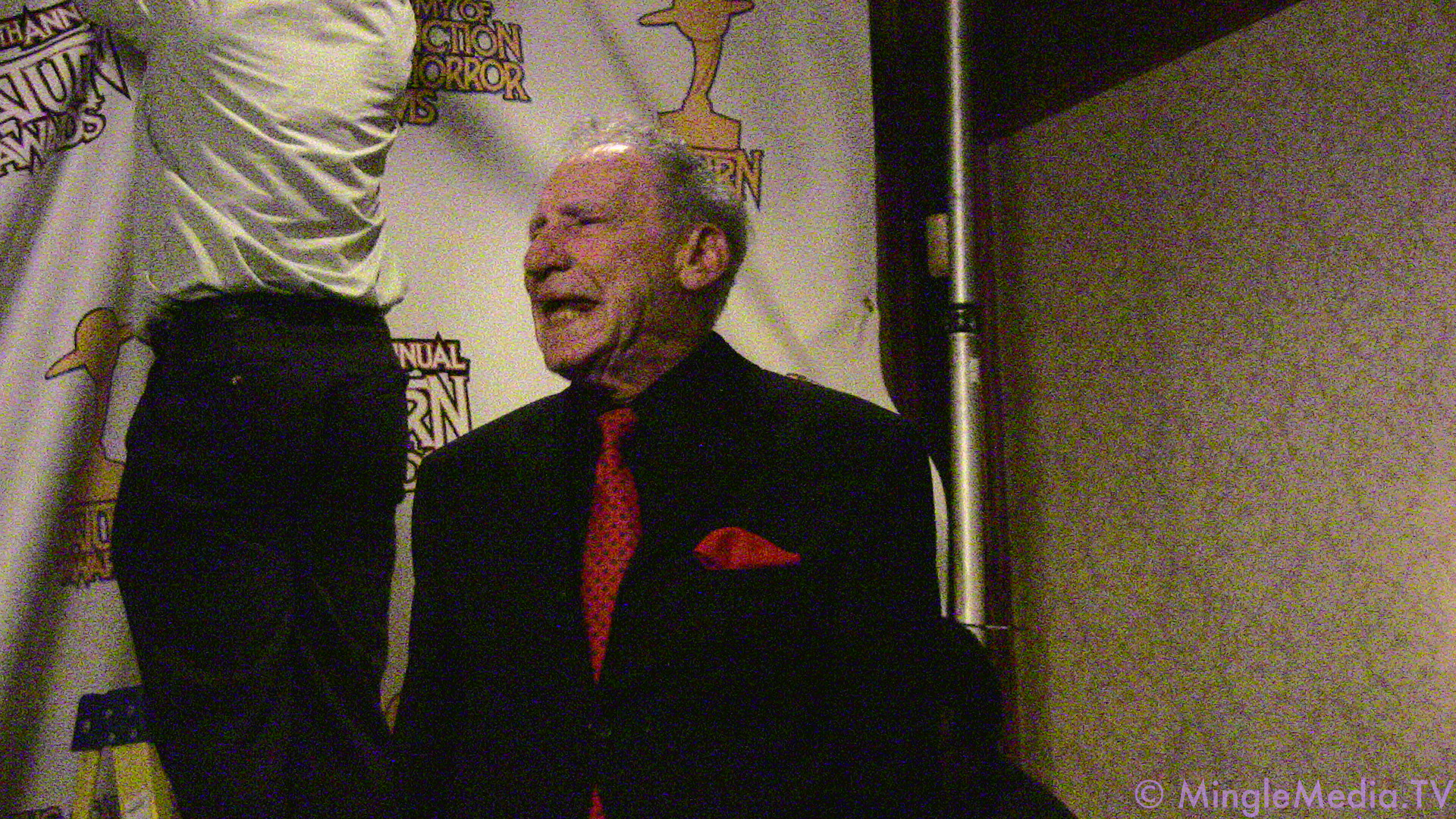The photograph captures a lively moment featuring the iconic comedian Mel Brooks. Dressed in a black suit with a bright red tie adorned with black dots and a matching red pocket square, Brooks, who has gray, balding hair, appears animated with his mouth open as if laughing or speaking energetically. The background on the left side is dark, transitioning to a multicolored wall with green and brown patterns towards the lower center. Behind Brooks, on the right side, hangs a white banner with indistinct yellow lettering, likely saying "Annual Awards Motion Horror." Assisting with the banner is a man in black pants and a white shirt, perched atop a yellow foot ladder. The image quality is grainy, and in the lower right corner, purple letters spell out "Mingled Media dot TV."